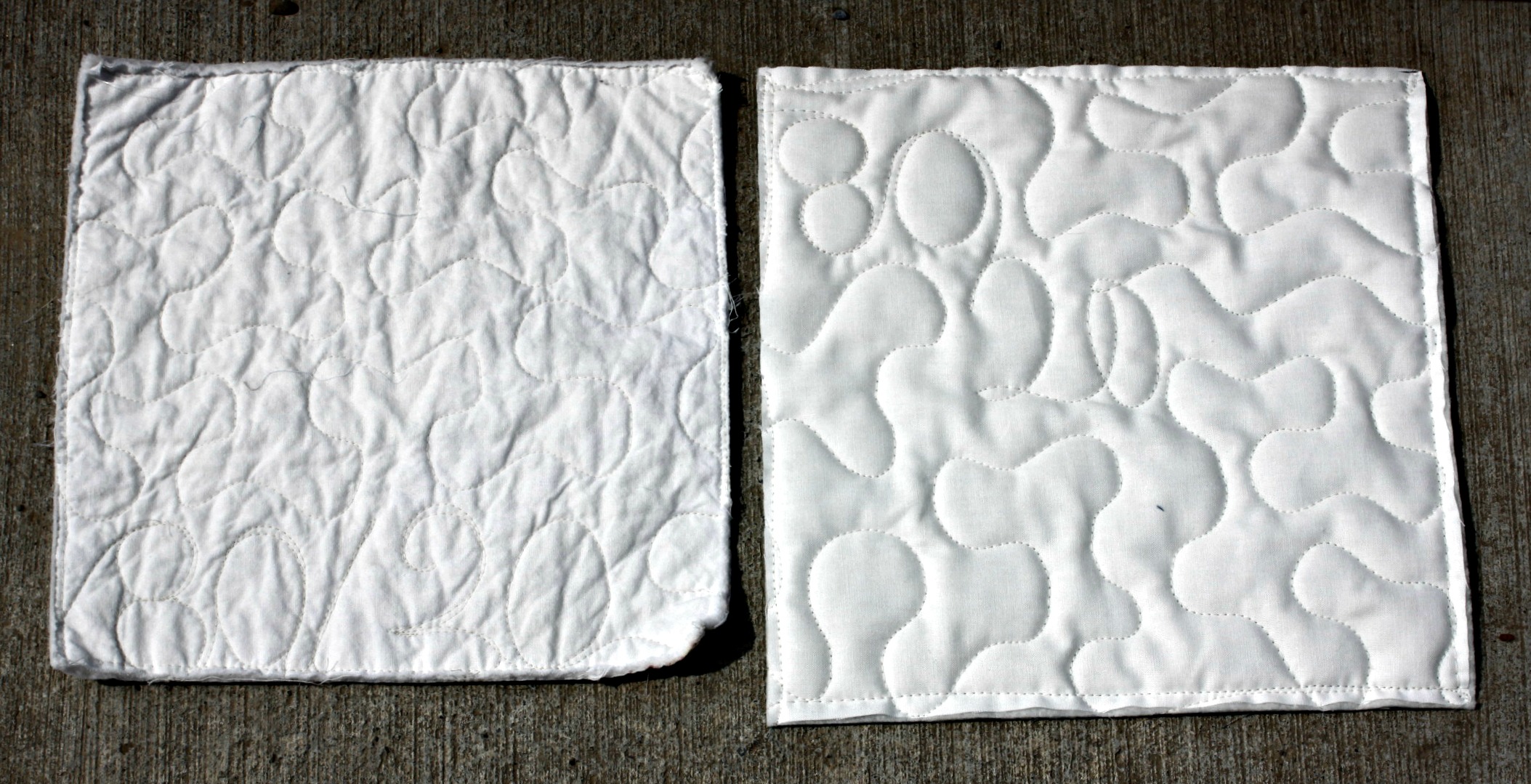The image features two square pieces of white cloth, likely used for household tasks like hot pads or napkins, positioned side-by-side on a tightly woven, dark gray carpet. The cloth on the left is smaller and visibly worn, with curled and slightly wrinkled corners, suggesting extensive use, washing, and drying. Its fabric is matted, and it has a swirly, stitched pattern that's somewhat broken down. The cloth on the right appears newer and slightly larger, with a similar but more intact raised design, and no significant wear or wrinkles. Together, these pieces of cloth illustrate the effects of time and use on fabric, while the backdrop of the gray carpet provides a neutral contrast that highlights the textures and conditions of the cloths.